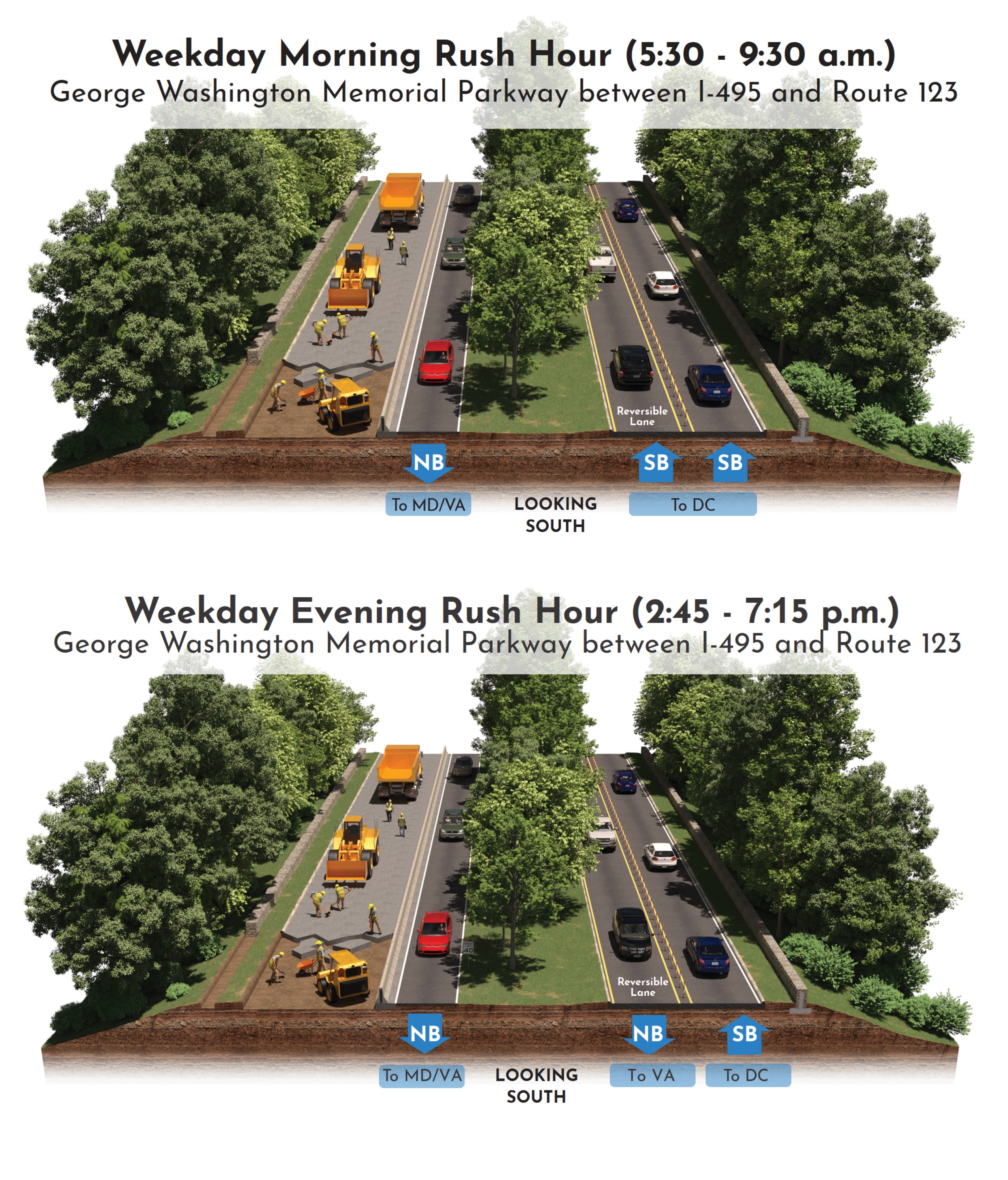The image showcases a detailed digital map or intricate mock-up of a specific area featuring traffic conditions during weekday rush hours on the George Washington Memorial Parkway between I-495 and Route 123. The map is split into two sections: the top part illustrates the morning rush hour from 5:30 to 9:30 a.m., while the bottom part shows the evening rush hour from 2:45 to 7:15 p.m. Both sections depict three rows of trees situated in grassy areas, separated by two roads each with two lanes. The left road is under construction, visible through the presence of yellow construction vehicles and workers laying concrete. Meanwhile, the right road displays normal traffic flow, with various cars including yellow tractor trailers, red, white, and black cars. Blue arrows indicate traffic directions, with labels such as “NB to N MD/VA” and “5b to DC” for the morning, adjusted to “NB to VA” and “5b to DC” for the evening. The images are rich with colors like blue, green, yellow, and gray, enhancing the detailed representation of the area and traffic conditions.